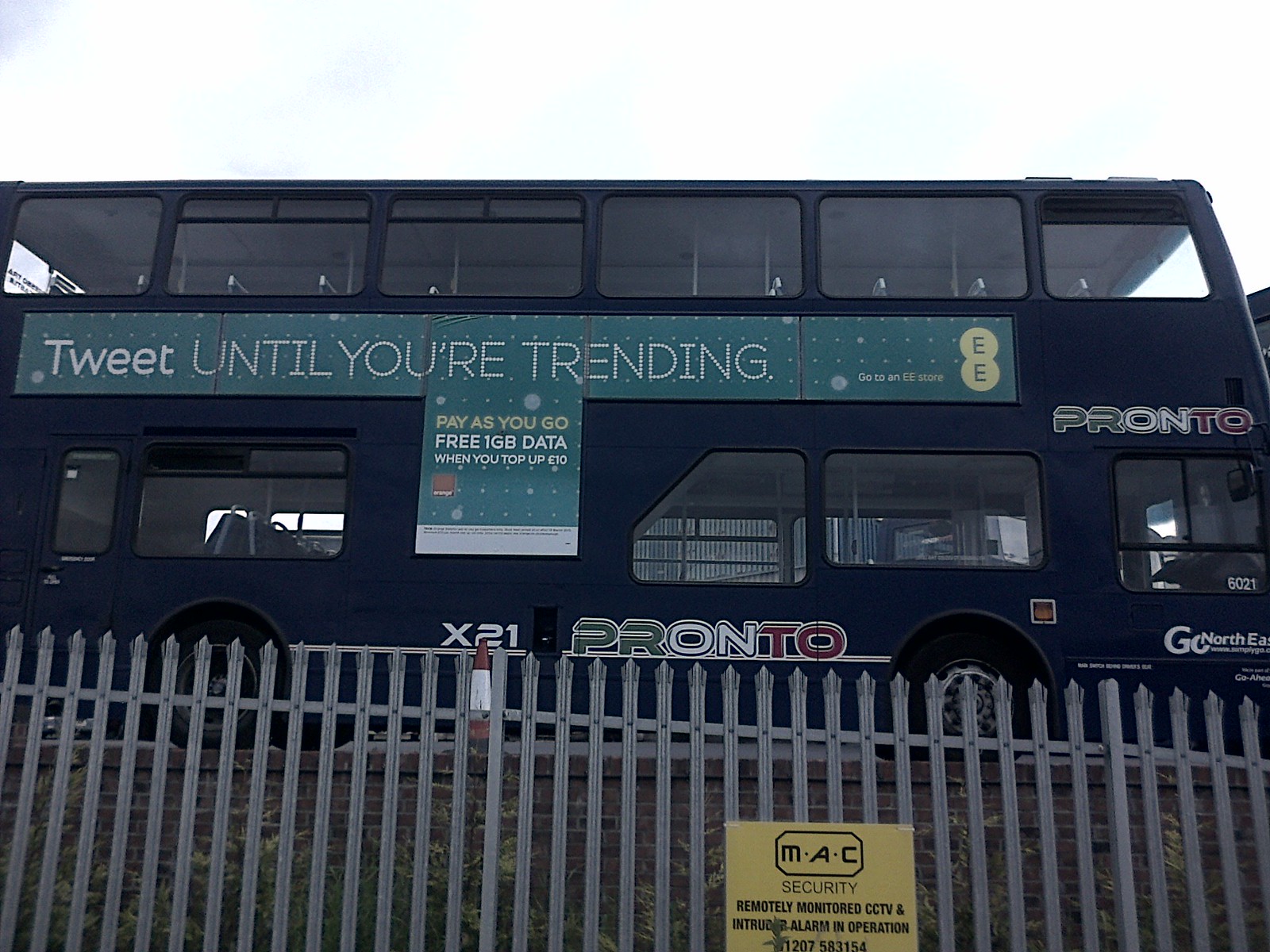This photograph showcases a dark blue double-decker bus prominently occupying most of the frame as it travels on the road. The bus, labeled "Pronto" with the route number "X21" visible, features large side windows spread across both its floors but appears empty as no passengers or driver are seen. Adorning its exterior in white letters is an advertisement that reads, "Tweet until you're trending - Pay as you go - Free 1GB data when you top up €10." The sky overhead is a pale white, enhancing the bus's vibrant color. In the foreground, there is a metallic green fence with a yellow and black warning sign indicating "Max Security - Remotely Monitored CCTV and Intruder Alarm in Operation." The fence borders a strip of grass along the sidewalk, where an orange and white traffic cone is also visible, adding further details to the scene.